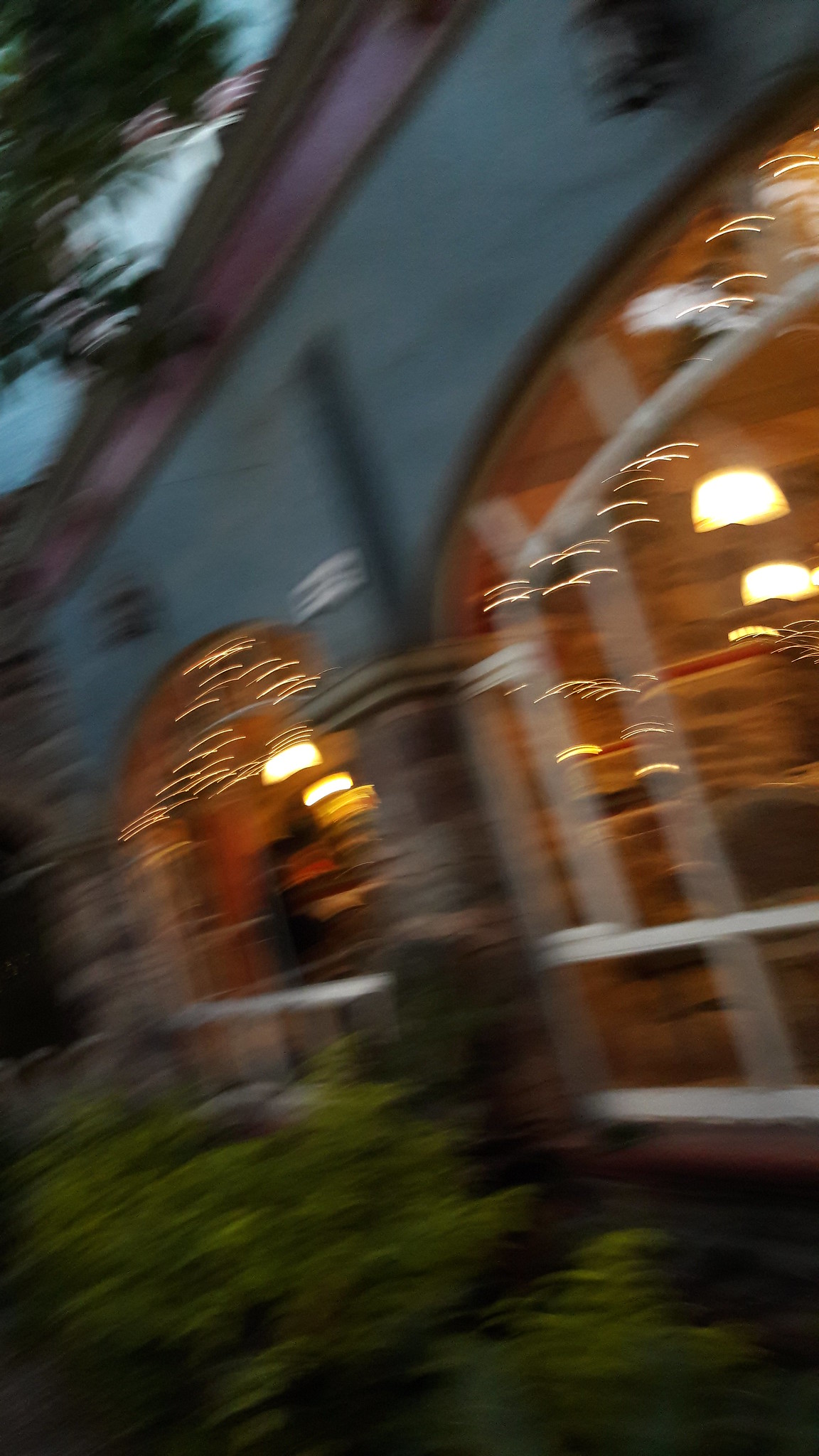This image is a blurry, vertically cropped color photograph captured during camera movement, resulting in streaks of light and an abstract composition. The central focus is the dynamic light emanating from within a building, potentially a restaurant, forming a series of squiggly lines that arc diagonally from left to right. These streaks display a spectrum of colors, predominantly white to yellow, with brighter orangish-yellow lights concentrated in the center.

The building features what appears to be an awning or arches, adding to the structure's intricate silhouette. In the lower foreground, patches of greenery are faintly visible, grounding the image in a natural element. The sky in the background adds depth and contrast to the vivid light trails. The photograph is angled such that the top of the building extends from the center-left to the upper-right corner, enhancing the composition’s dynamism. A vibrant blend of blues, oranges, and greens dominates the color palette, creating a visually striking scene.